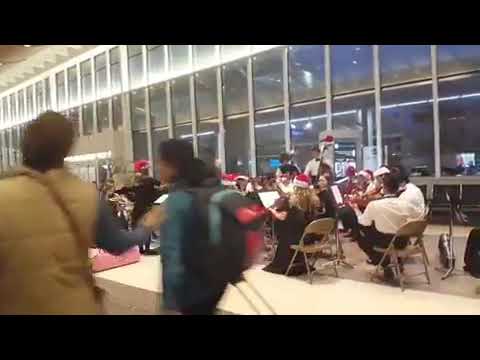This image captures the interior of a large room, possibly an airport, characterized by a far-left wall made entirely of a grid of windows, suggesting it's nighttime as darkness is visible outside. The scene is reminiscent of the 70s or 80s due to the grainy and low-detail quality of the image. The floor below is a patchwork of white, brown, and gray tiles, adding to the vintage ambiance. 

In the background, a symphony or band is seated in gray and brown metal folding chairs, playing various instruments—including violins, violas, and a stand-up bass. The musicians are dressed in black and white outfits and many are wearing red-and-white Santa hats, indicating that the photo was taken around Christmas.

The focus is primarily on the symphony, but in the foreground, slightly blurry, are two individuals walking by. One person, wearing a black and teal coat and a backpack with black, red, and teal colors, is identifiable as an Indian woman with her hair pulled back. Another figure nearby is seen with a tan coat, gloves, and a bag strap extending from their left shoulder to their right hip. The overall environment suggests a bustling yet organized setting, with the musical performance adding a festive atmosphere to this expansive indoor space.